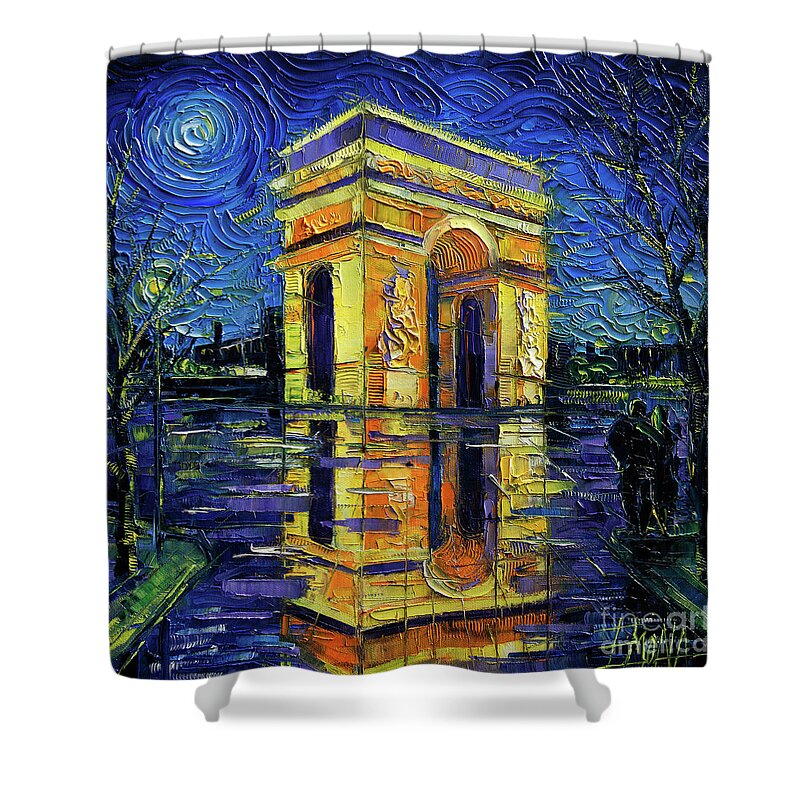The image is a detailed Impressionist painting depicted on what appears to be a shower curtain or a textile canvas, hanging from a curved white pole with shower curtain rings. The top part of the image features a darker blue, textured sky with swirling brushstrokes, reminiscent of Vincent van Gogh's "Starry Night." Below the sky, a body of water, like a pond or river, reflects the scene above it.

At the center, there is a large, rectangular structure resembling the Arc de Triomphe in Paris. The monument has a flat roof and a prominent arched gateway in the middle, allowing one to see through it. The structure is adorned with hues of yellow and orange, standing out against the predominantly blue surroundings. 

The landscape includes black-painted trees on either side and patches of green scattered across the land. Notably, the entire scene is mirrored in the water below, enhancing the painting's depth and reflective quality. 

In the bottom right corner, there is a dull grey watermark that says "fine art," accompanied by the artist's signature below it. The whole painting has a distinct textured finish, reflecting the Impressionist style, with dynamic and expressive brushstrokes.